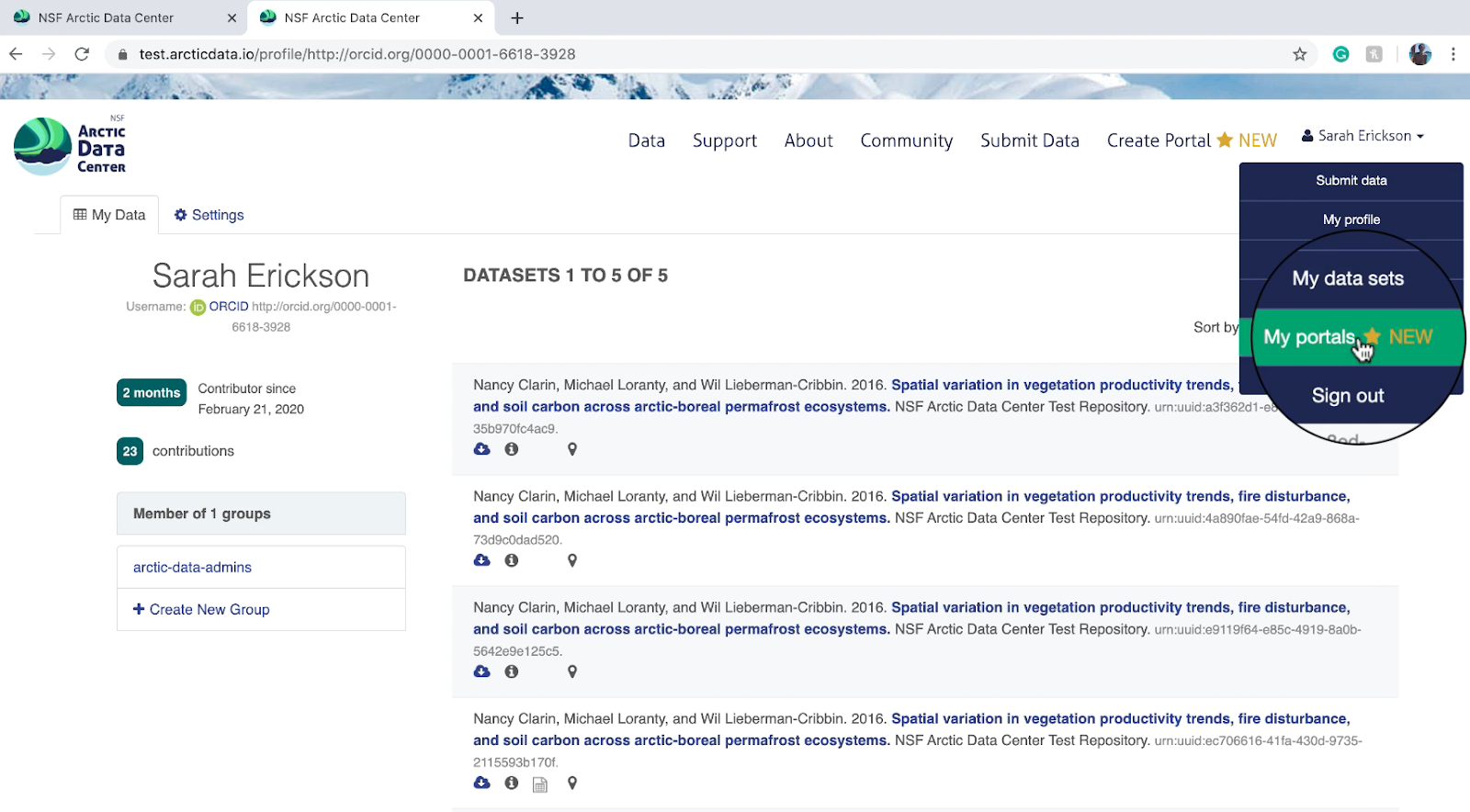A detailed screenshot of a Chrome browser displaying two open tabs, both on the NSF Arctic Data Center website. The website features a clean white background with a prominent top navigation bar. Positioned at the top left is the Arctic Data Center logo, consisting of text "Arctic Data Center" beside a circular icon depicting what appears to be auroras in the sky above snowy ground.

The navigation menu is centrally and right-aligned, featuring buttons labeled 'Data', 'Support', 'About', 'Community', 'Submit Data', and 'Create Portal' with a star icon indicating its novelty. Additionally, there is a drop-down menu labeled 'Sarah Erickson'. When expanded, this drop-down reveals a blue box with options for 'Submit Data', 'My Profile', 'My Datasets', 'My Portals' (highlighted with a magnified circular overlay and a hand cursor), and 'Sign Out'.